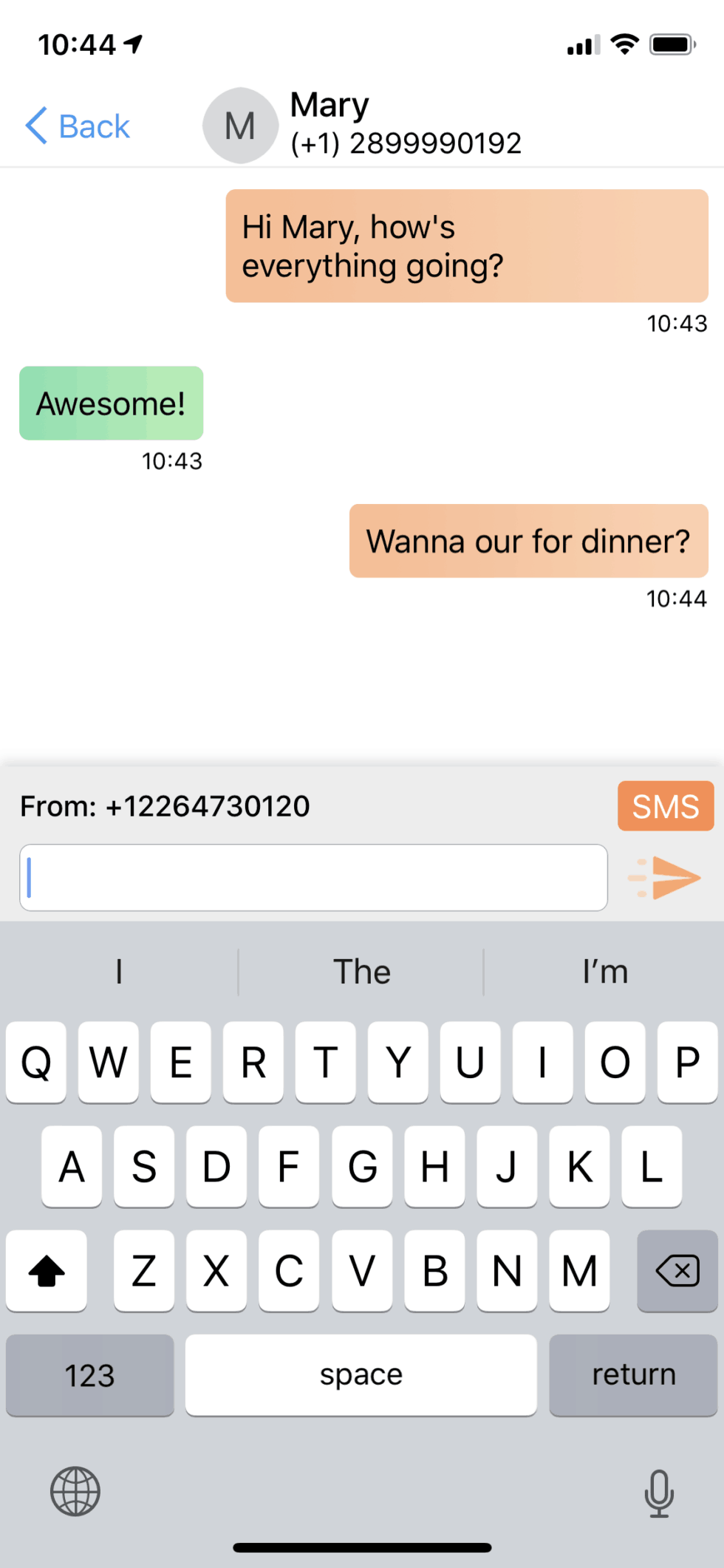A detailed caption for the phone screenshot:

---

The screenshot displays a smartphone interface with various elements. In the top-left corner, the time is shown as 10:45 with a small black arrow button next to it. The top-right corner contains three icons for signal strength, Wi-Fi, and battery level, all depicted in black.

Below this is the messaging app interface. Centered at the top is the contact name, "Mary," represented by an "M" icon within a circle. Next to her name is a notification indicating one unread message (1), followed by her phone number, (289) 999-0192. On the left-hand side, there is a blue back button with an arrow.

The conversation thread is displayed below. The first message, in orange text, reads, "Hi Mary, how's everything going?" Mary’s response, displayed in green text, is "Awesome." Another orange message follows, stating, "One hour for dinner."

At the bottom of the screen, there is a text input field with the keyboard pulled up. The field shows the placeholder text "From" with an adjacent SMS button and a space to input the sender's name. The visible keyboard includes all the standard keys such as letters, space bar, return key, and a number pad.

---